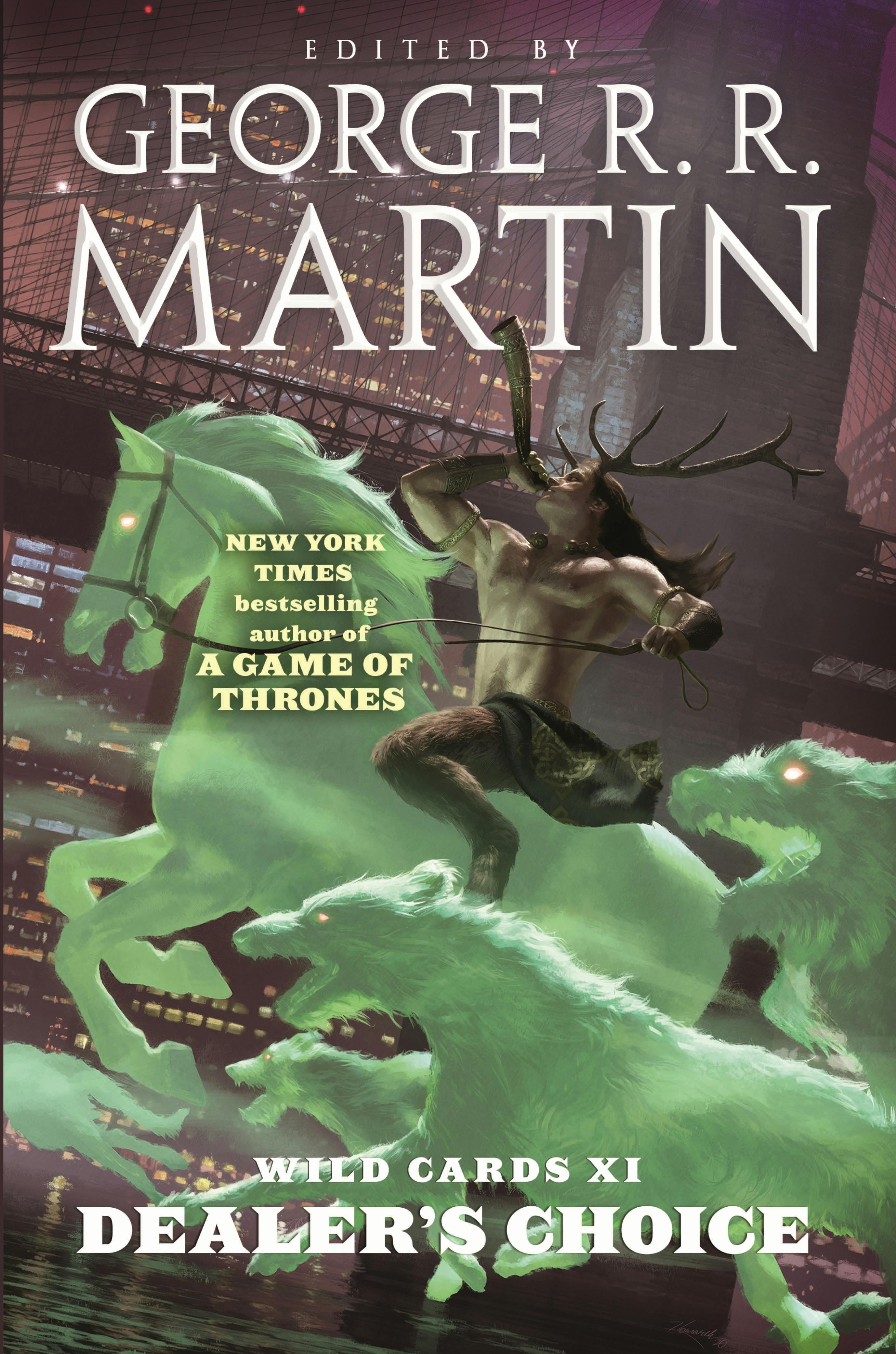The book cover for "Wild Cards 11: Dealer's Choice," edited by George R.R. Martin, New York Times bestselling author of "A Game of Thrones," features an urban nightscape backdrop with a bridge and a lit-up skyscraper. In the foreground, a satyr-like figure with goat legs, antlers, and a bare torso blows a power horn while riding a ghostly green horse. Surrounding him are four hairy wolves with glowing eyes, all racing towards the left. The title "Wild Cards 11" is prominently displayed at the bottom, emphasizing the fusion of fantasy elements and an urban setting.